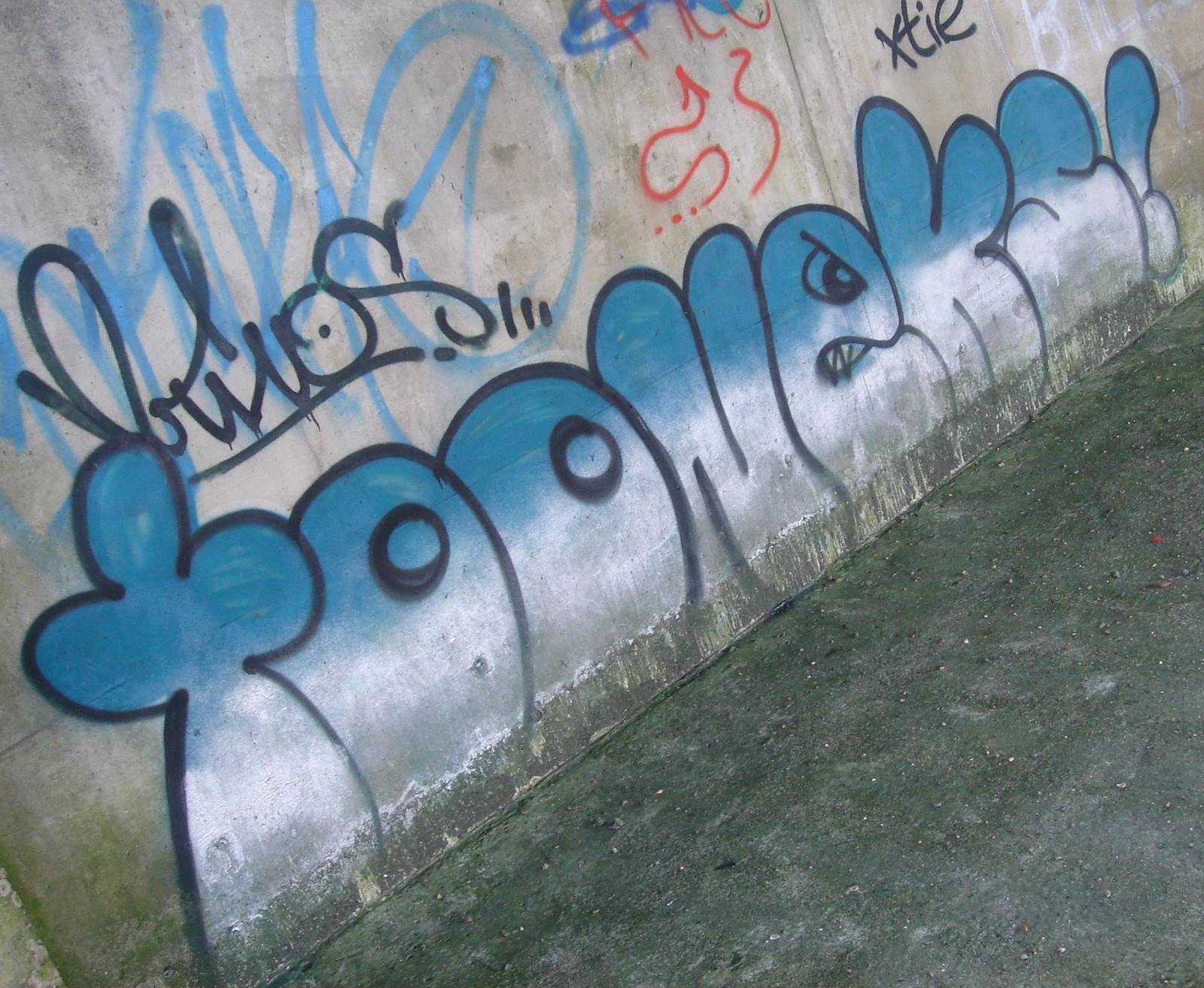This is a photograph of a light gray, slightly faded stone wall covered in assorted graffiti. Shot at a three-quarter angle, the image shows the wall running diagonally from the lower left center to the upper right, meeting a darker gray concrete sidewalk at the base. The ground is littered with small pebbles and paint splatters, indicating frequent graffiti activity. Prominently, the word "TOONEKS" is spray-painted in large, cartoonish bubble letters across the wall’s bottom section. The letters transition from a blue hue at the top to a lighter white and finally to a light gray at the bottom. Above this word, smaller graffiti in black marker-like strokes, light blue paint scribbles, and two curving red lines add layers of intricate street art. To the right, faded black graffiti, possibly spelling out "XTI" or "XFIE," merges with the colorful chaos. The detailed layering suggests a vibrant yet cluttered urban canvas, captured in the clear light of day.